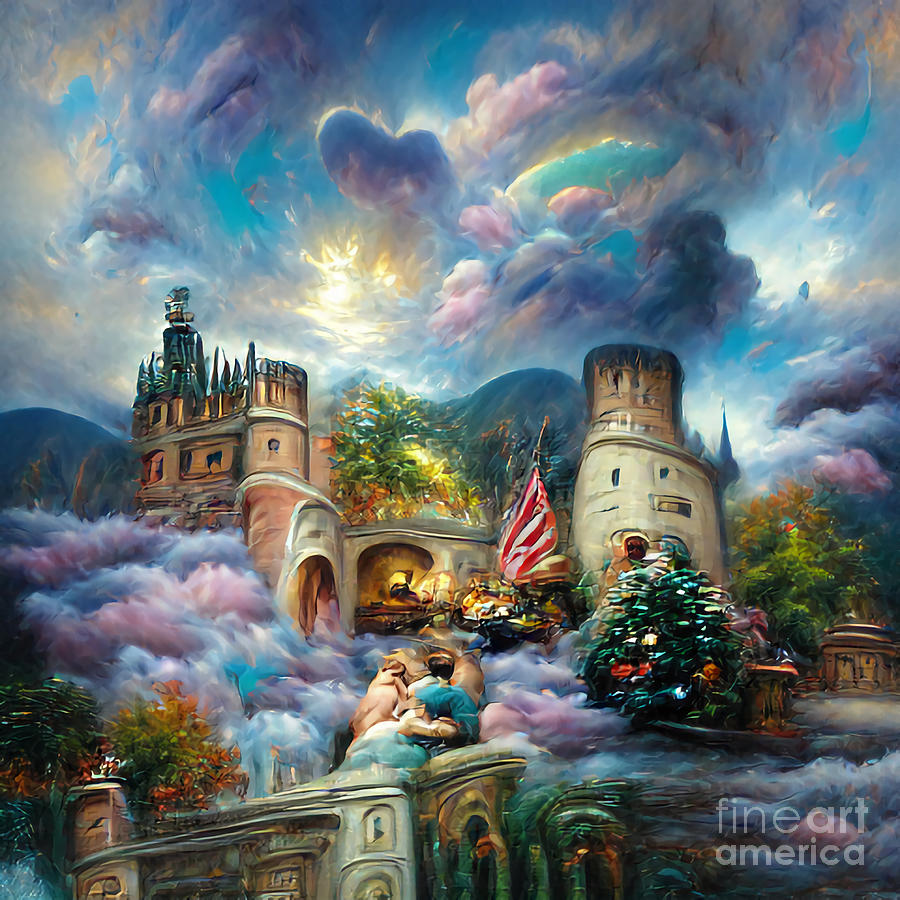This vibrant digital painting, possibly AI-generated, features a fantastical castle nestled on a hill at the foothills of towering mountains, with some abstract figures and a building in the foreground. The castle is adorned with impressive trees and plants bearing enormous flowers, and it has striking lamps and lights that add a magical touch to its appearance. A flag with red and white stripes flutters between the castle towers, complemented by a river-like formation of pink, blue, and white clouds swirling around its base, resembling a flow of cotton candy. The sky above is a dazzling array of pink, purple, teal, turquoise, yellow, violet, and white, with luminous swirly clouds that blanket the entire scene. A dramatic light source, possibly behind the clouds, illuminates the sky and creates a billowing storm effect near the mountains. The lower right corner of the image is marked with "Fine Art America," indicating the artwork's origin.